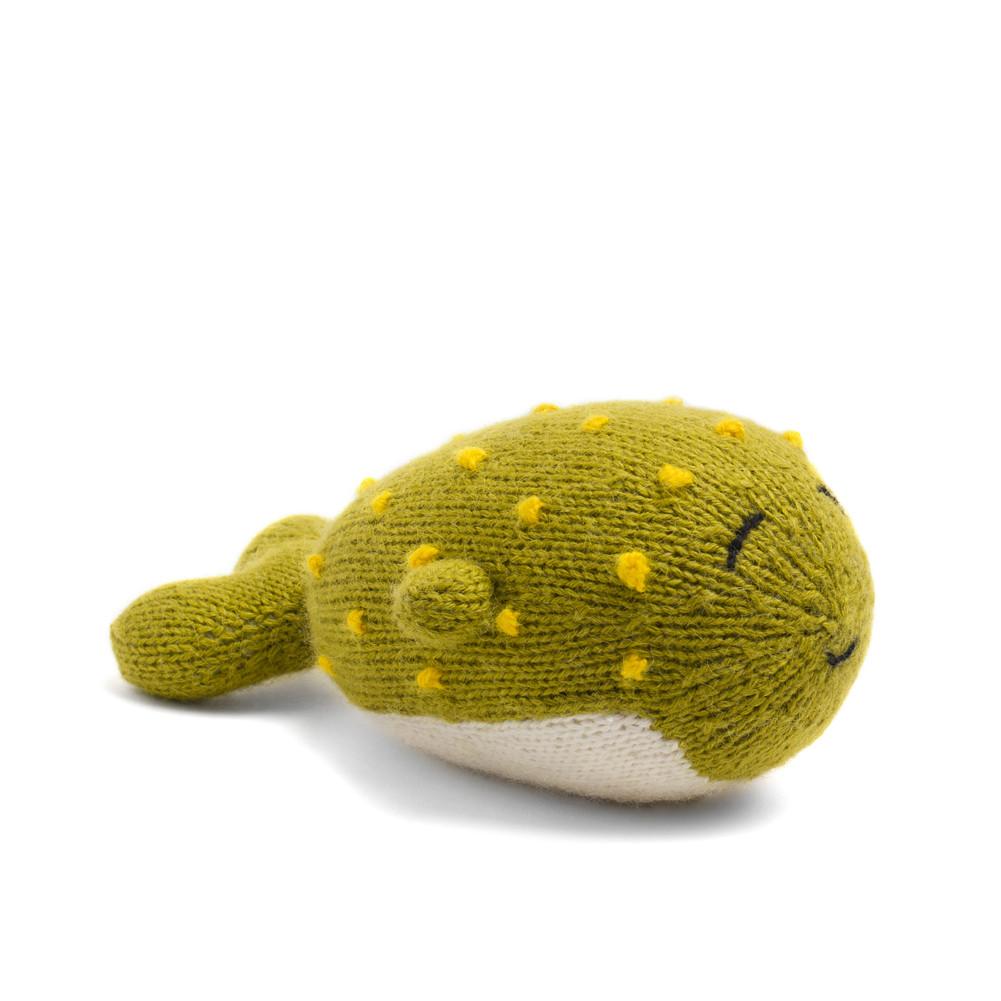The image showcases a small, intricately knitted stuffed toy that resembles a cheerful blowfish. The blowfish features an olive green upper body that transitions into a white underbelly. Its design includes subtle, black stitched slits for eyes and a delicate, embroidered smile. The body is adorned with raised yellow yarn dots, mimicking the texture of a blowfish's spines. Small circular fins protrude from its sides, and a small, heart-shaped tail fin extends from its back. The toy is crafted from knitting material, possibly resembling a sock texture, and appears cozy and soft. Photographed against a white background with a faint shadow, the image emphasizes the toy's charming and happy demeanor.